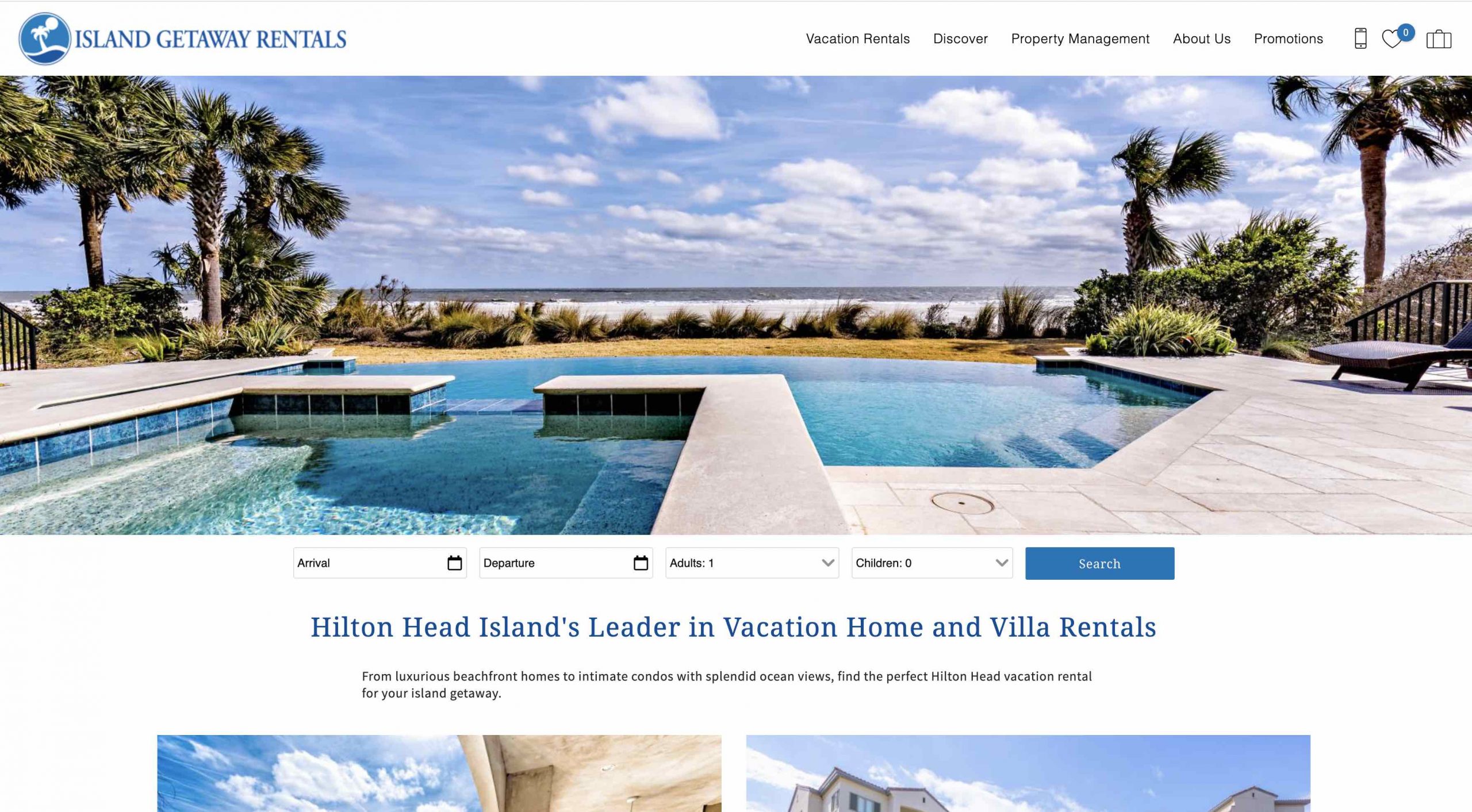This image features a pristine white background with a prominently placed header that reads "Island Getaway Rentals." Adjacent to the header is a blue circular logo depicting a beach scene with palm trees. The navigational menu includes options such as Vacation Rentals, Discover, Property Management, About Us, and Promotions. In the top right corner, there are icons indicating battery status, a heart symbol, a notification circle with the number three, and a small suitcase. A blue line runs across the top of the image for added visual clarity.

Dominating the center of the image is a stunning photograph of a luxurious beachfront getaway. The focal point of the photograph is a large, inviting pool, accompanied by a breathtaking beach adorned with lounge chairs and swaying palm trees. Below this, there is a user interface section that allows for the entry of arrival and departure dates, the number of adults and children, and features a prominent blue "Search" button.

Further down, text highlights that the property is recognized as Hilton Head Island's leader in vacation home and villa rentals, with additional descriptive information provided. The bottom portion of the image includes partial views of two related photographs, alluding to more beautiful vacation options.